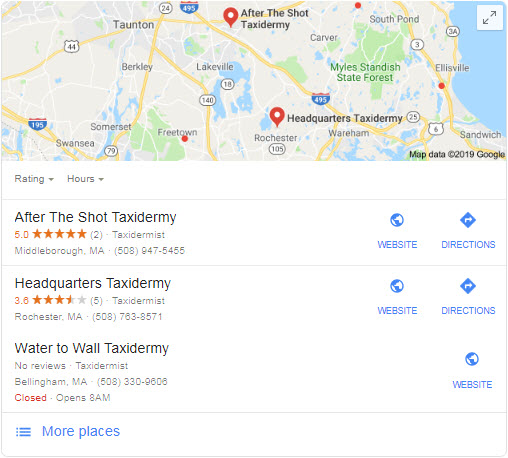This is a detailed screenshot taken from Google Maps. The upper third of the image displays a map. The land is depicted in a tan color, extending from the left to about an inch from the right edge of the image. In the center of the map, there is a small blue area representing a lake. Along the right side, approximately two inches from the top right corner to near the bottom right corner, there is more blue representing a body of water. Yellow lines indicate the interstates, while white lines mark other roads. 

In the bottom left, about an inch from the edge, there is a green area, signifying a park or forest. Another green area is located to the left of the body of water on the right, marking the "Mild Standard State Forest." The map also features two red pins: one positioned in the top center and the other in the bottom center. 

Below the map is a white-bordered section which includes a ratings and hours dropdown tab, followed by a thin dividing line. The bold black heading reads "After the Shot Taxidermy," accompanied by a five-star rating. Below this, in quotations, it says "Taxidermist." Further details include the address and phone number. On the right side, there is a globe icon labeled "Website," and below it is a directions icon labeled "Directions."

Following this is information for "Headquarters Taxidermy," including the rating, address, and the same right-hand icons. Below this, "Water to Wall Taxidermy" is listed; it has no reviews and states "Taxidermist," providing the location and phone number. This entry is marked in red as "Closed - opens 8 AM." Though there is no directions icon here, there is a website icon labeled "Website."

In the bottom left corner of the screenshot, there are sideways exclamation marks pointing left, and a blue link labeled "More places."